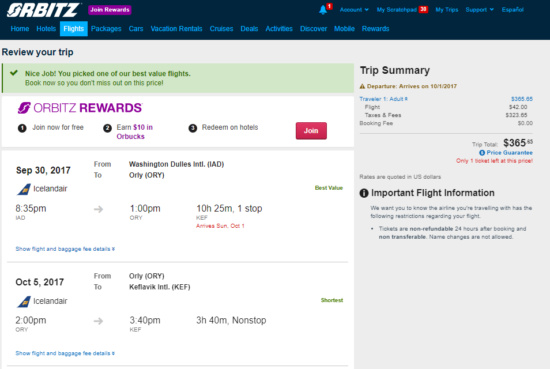In this image, we see a screenshot of a travel website, Orbitz, with several distinct elements despite the image being very blurry. At the top, there's a dark blue bar, approximately an inch thick, spanning the width of the screen. On the left side of this bar, the Orbitz logo is displayed in white. Adjacent to the logo, there's a pink "Join Rewards" button. Further to the right, slightly blurred, are icons and text for notifications, account management, and additional options like "My Trips," "Support," and "Español."

Beneath this bar, on the left, the tabs "Home," "Hotels," "Flights," "Packages," "Cars," "Vacation Rentals," "Cruises," "Deals," "Activities," "Discover," "Mobile," and "Rewards" are listed horizontally, indicating the navigation menu.

On the left side of the screen, under these navigation tabs, there is a section labeled "Review Your Trip," suggesting that a user is in the process of booking or reviewing travel plans. The website promotes the Orbitz Rewards program, offering a $10 bonus for joining. The details of the trip are specified, with a departure on Iceland Air scheduled for September 30, 2017, at 8:35 PM, arriving at 1 PM. The return flight is set for October 5th. 

On the right side, there is a "Trip Summary" section displaying the total price for the trip, which is $365.